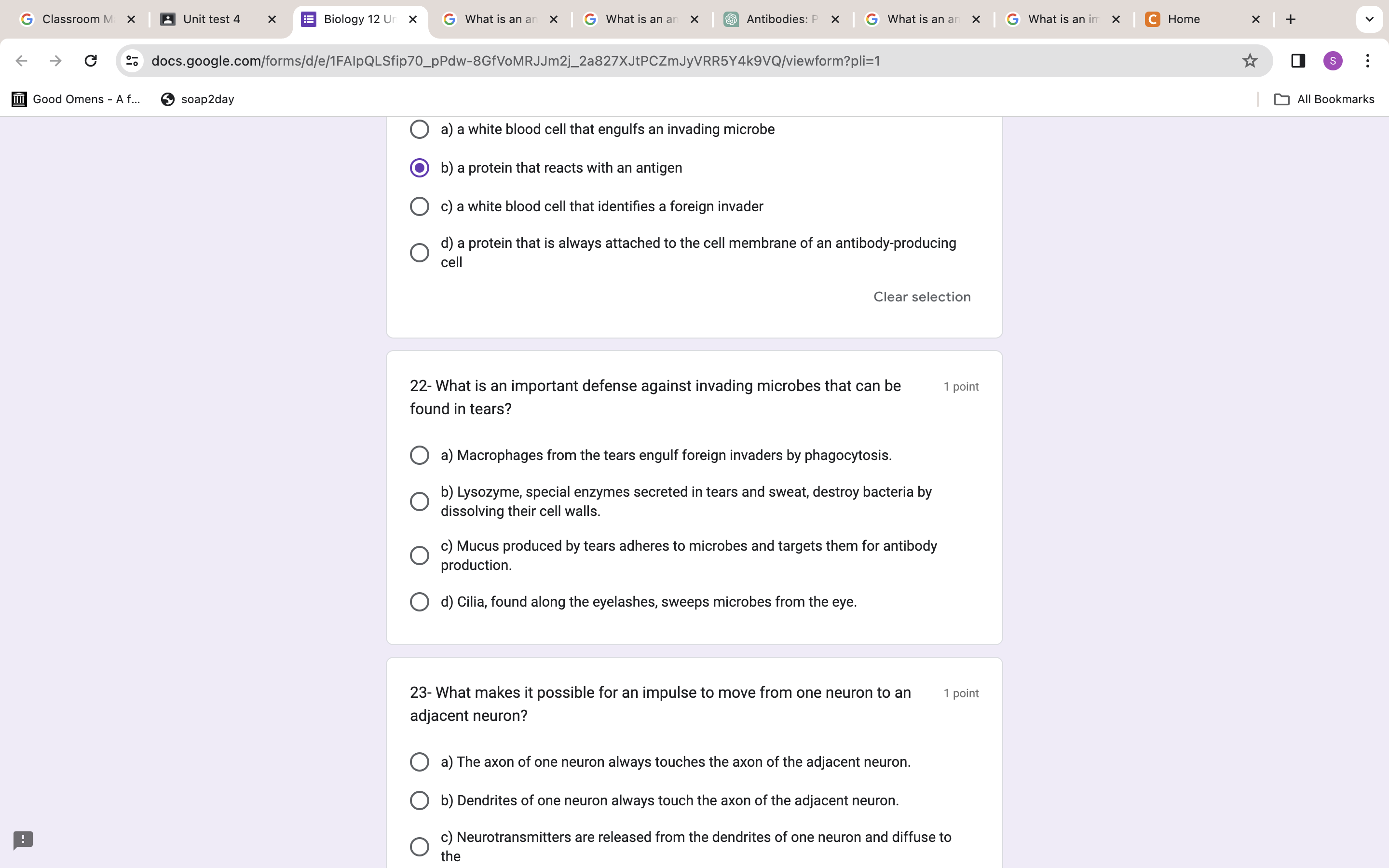The image appears to be a snapshot of an academic website or online classroom platform. At the top of the page, there is a grey bar extending across the screen, resembling a row of tabs commonly used in web browsers or online course management systems.

From left to right, the first tab features a white circle with the Google "G" icon, followed by the label "Classrooms" in black text. The next tab is a black box with a white silhouette of a person and the label "Unit Test 4" in black text. Following this is a highlighted tab with a purple box labeled "Biology 12."

Continuing to the right, there is another tab with a white circle containing the Google "G" icon and partially visible text that begins with "What is a" but becomes blurry. This pattern repeats with two more tabs, each with the Google "G" icon and similarly obscured text.

Further along, a green box with white text labeled "Antibodies" is followed by yet another series of white circles with the Google "G" icon and blurred text. The last tab in this sequence is an orange box with a white "C" and the label "Home."

Below the grey bar, there is a search bar with the URL "docs.google.com" and a web address. On the left-hand side of the page, there is a black box labeled "Good Omens" and an adjacent black icon of a globe with the text "Soap Today."

The main content area seems to be part of a quiz or test. There is a white circle next to the statement "A white blood cell that engulfs an invading microbe," followed by a purple circle (suggesting it has been selected) with the text "B. A protein that reacts with an antigen." Below these, another white circle precedes the text "C. A white blood cell that identifies a foreign invader," and another white circle follows with the text "D. A protein that is always attached to the cell membrane of an antibody-producing cell."

Further down, a separate box is labeled "22," accompanied by the question, "What is an important defense against invading microbes that can be found in tears?" Below this question, four empty circles await selection of the correct answer from choices labeled A, B, C, and D.

Lastly, another white box marked "23" poses the question, "What makes it possible for an impulse to move from one neuron to an adjacent neuron?" with answer options A, B, and C waiting to be selected below.